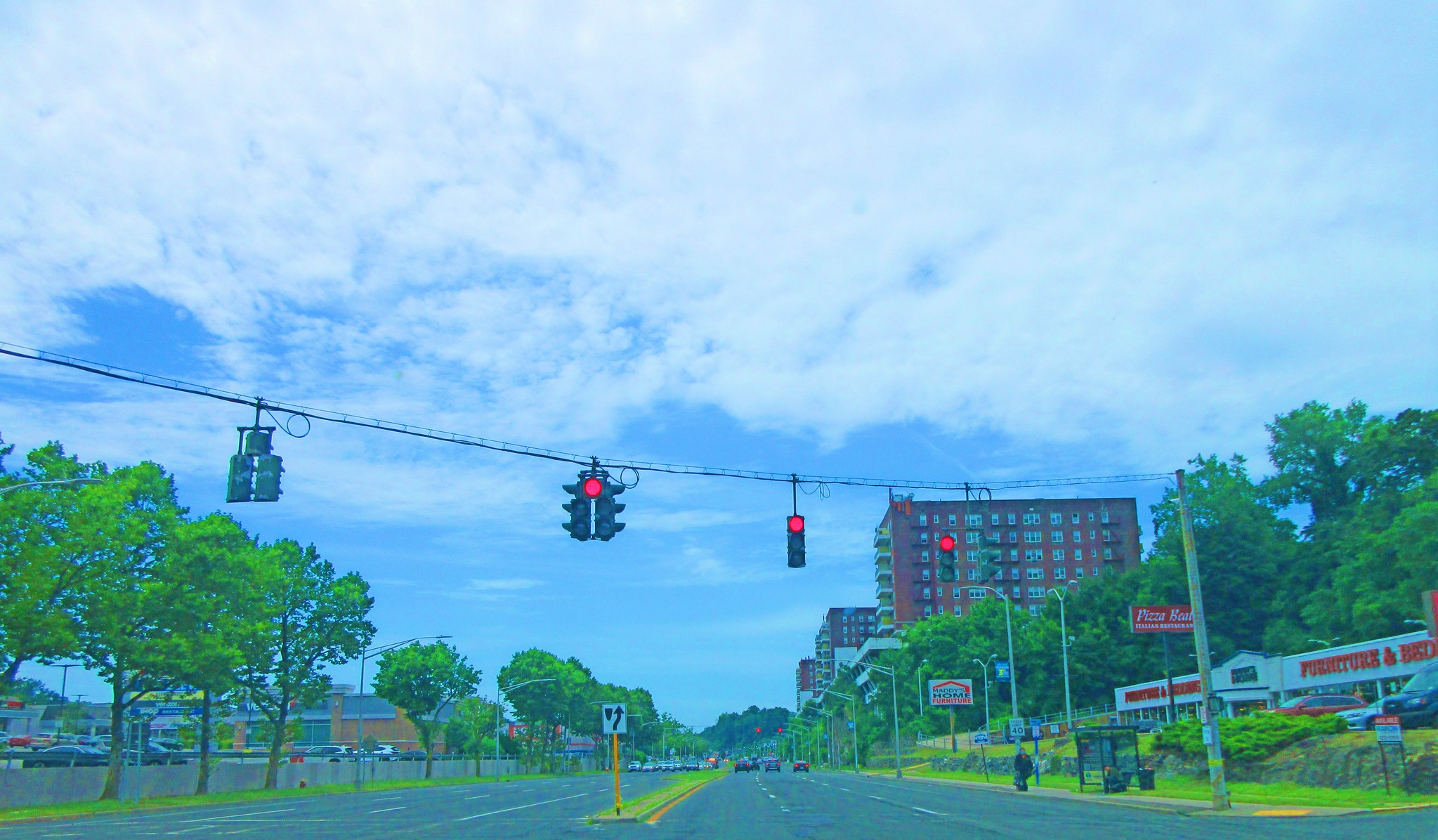This is a color photograph depicting an urban street scene, with an overall unnatural blue and green tint, possibly from a filter or as an AI-generated image. In the foreground, there are roads flanking a thin strip of grass that features a small rectangular object, potentially a parking meter. Overhead, a series of traffic lights spans the street, with three in the center displaying red signals and one additional light on the left.

Trees with lush green leaves line both sides of the road, providing a natural border to the urban environment. On the left side of the image, several cars are parked in front of a building. To the right, three tall buildings dominate the scene. The foremost building is notably tall, featuring brown walls punctuated by numerous small, square grey windows. Adjacent to this on the far right is a smaller structure topped with a red sign bearing an unreadable inscription. A red street sign is visible above this building.

The sky exhibits a gradient, transitioning from blue at the bottom to grey clouds at the top, adding to the scene's overall contrast and complexity.